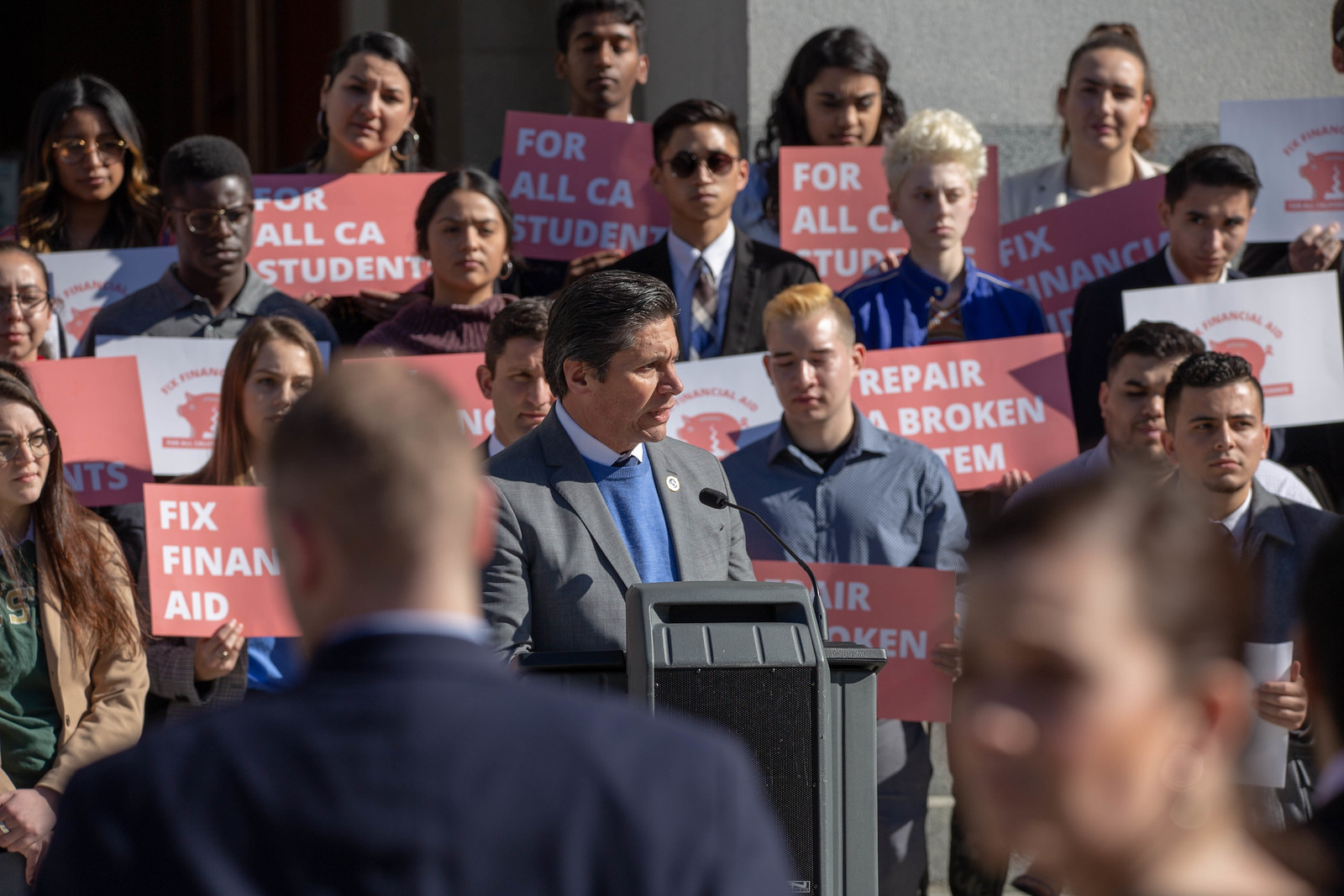This is a photograph taken outdoors, capturing a man giving a speech at a black podium. The man is dressed in a white shirt, a blue sweater, and a black coat, with his hair neatly combed back and a serious expression on his face. Speaking into a microphone, he stands at the front and center of a group of approximately 18 young people who appear to be students. These students are holding various signs—some pink, some white, some with red writing, and others depicting the California bear symbol. The text on the signs includes messages like "Repair a Broken Item", "Fix Financial Aid for All California Students", and "Repair the Broken System". Behind the speaker and students is the wall of a building, while blurred images of heads in the foreground indicate the presence of an audience, suggesting that this is a student rally or protest advocating for improvements in financial aid and educational resources in California. The scene is well-lit, highlighting the peaceful and organized atmosphere of the event.